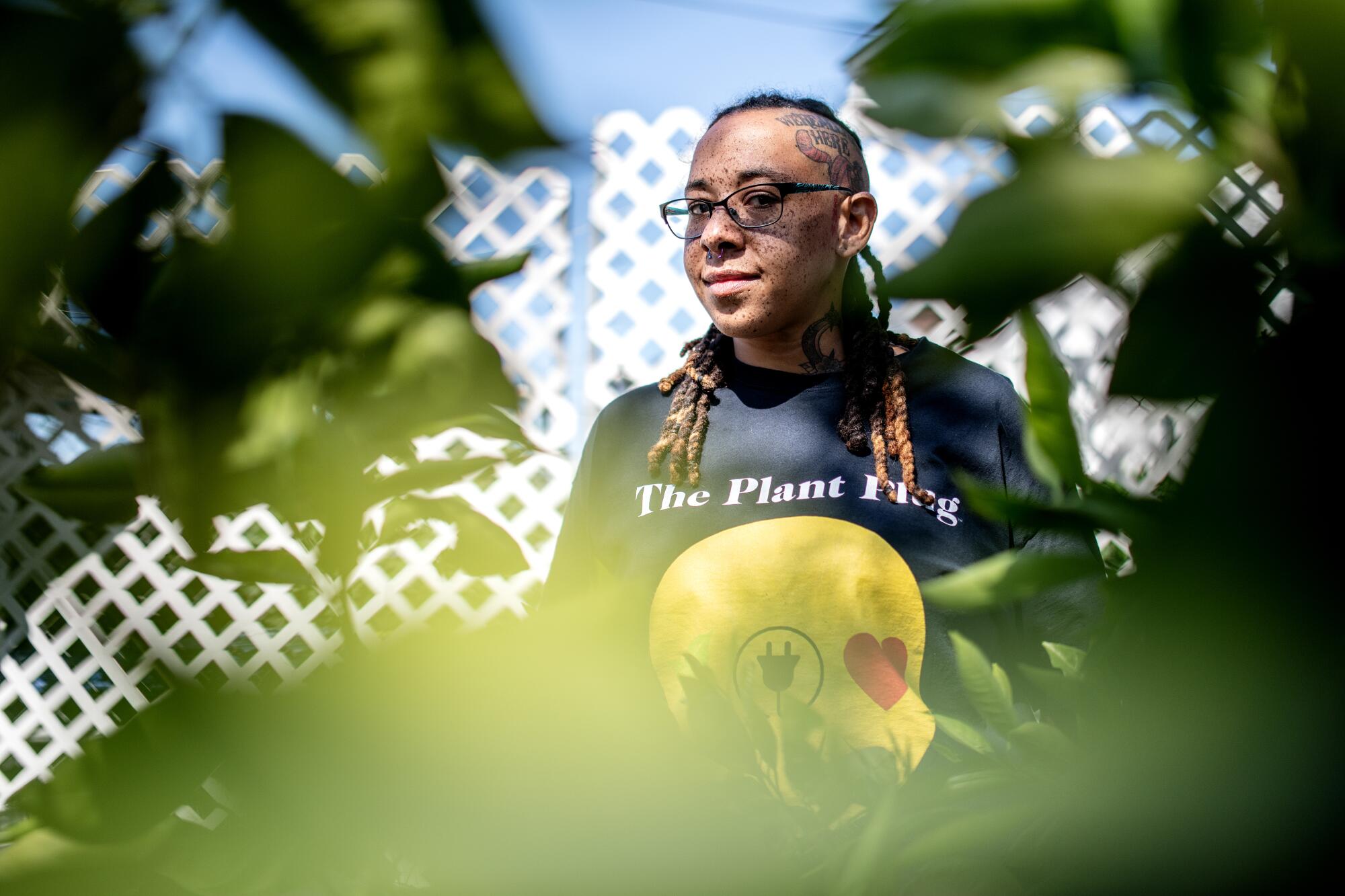This photograph features an African American woman with distinctive features and a thoughtful expression. She has brown dreadlocks that extend to her chest, with the left side of her head shaved to reveal a tattoo. The tattoo is partially readable and includes the word "HERE" along with some design elements. She sports clear glasses with black frames and has a face dotted with numerous freckles. The woman is dressed in a black long-sleeved shirt that bears white lettering stating "the plant," though the final word is obscured by her hair. A yellow circle with an electrical plug inside it and a red heart to its right is prominently displayed on her shirt. The background showcases a white lattice fence leaned against a blue wall, and the shot is taken through a blur of green leaves, giving a sense of someone observing from a hidden vantage point.